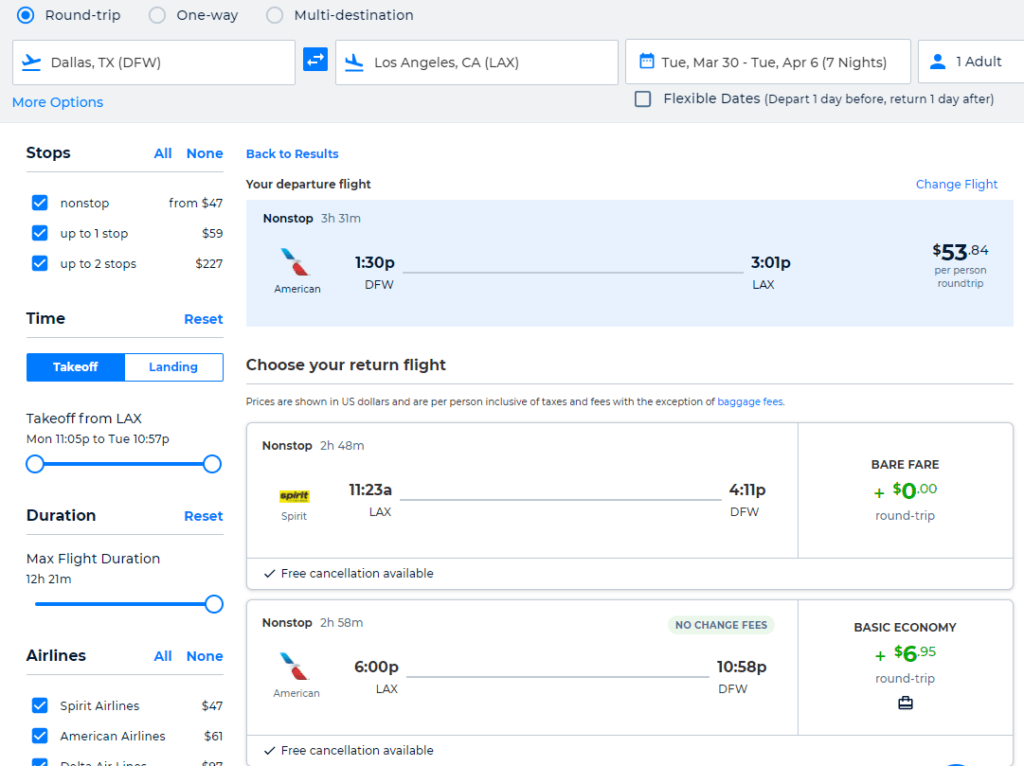A screenshot of a webpage displaying a window with detailed information on airline tickets. The window features a clean, white background and is organized into multiple sections. In the upper left corner, a blue radio button is highlighted, indicating the 'Round Trip' option. Adjacent to it are radio buttons for 'One-Way' and 'Multi-Destination' options. Directly below these radio buttons, there are four small search bars that display various airlines, forming the main frame at the top of the image. Beneath this main frame, the webpage is further divided into three horizontal sections. To the left of these sections, there is a vertical frame containing filter options, written in black. The options listed include 'Stops', 'Time', 'Duration', and 'Airlines'.